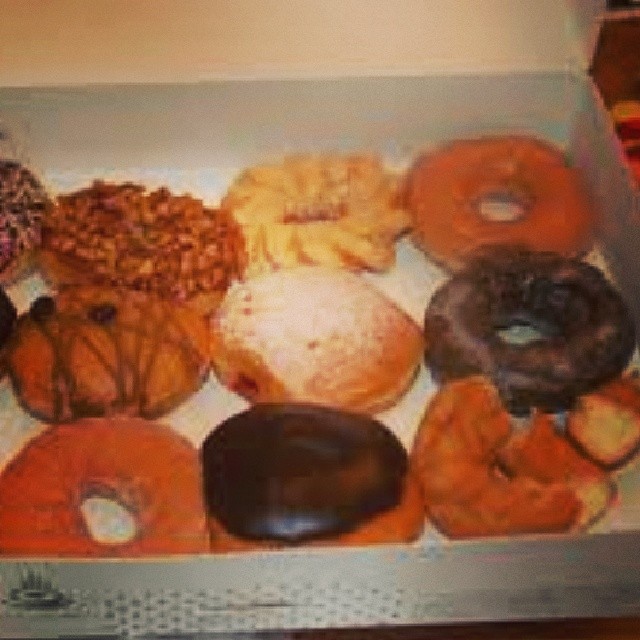This square, fuzzy, and grainy photograph appears to be taken with a low-quality digital camera or uploaded at very low resolution. It captures an open white donut box, likely from a well-known chain like Dunkin' or Krispy Kreme, evidenced by a steaming cup of coffee logo on the side, although the exact branding is unclear. The interior of the box holds a variety of donuts organized in an assumed 4x3 grid, with nine clearly visible and part of a tenth peeking in from the left. 

The donuts include a mix of types: plain, tan-colored rings with holes, a solid donut with chocolate frosting, and another chocolate glazed donut with a hole. Amidst them are a cruller, a powdered jelly donut, and a Boston cream with chocolate glaze. One donut appears partially broken into three pieces at the bottom right corner. The lighting creates a warm orangish glow, hinting at tungsten illumination. Texture-wise, most donuts present smooth surfaces, with occasional toppings like sprinkles, nuts, and a striping pattern observable on a few, enhancing their visual diversity. The overall clarity is low, but the assortment and arrangement of the donuts are distinguishable.